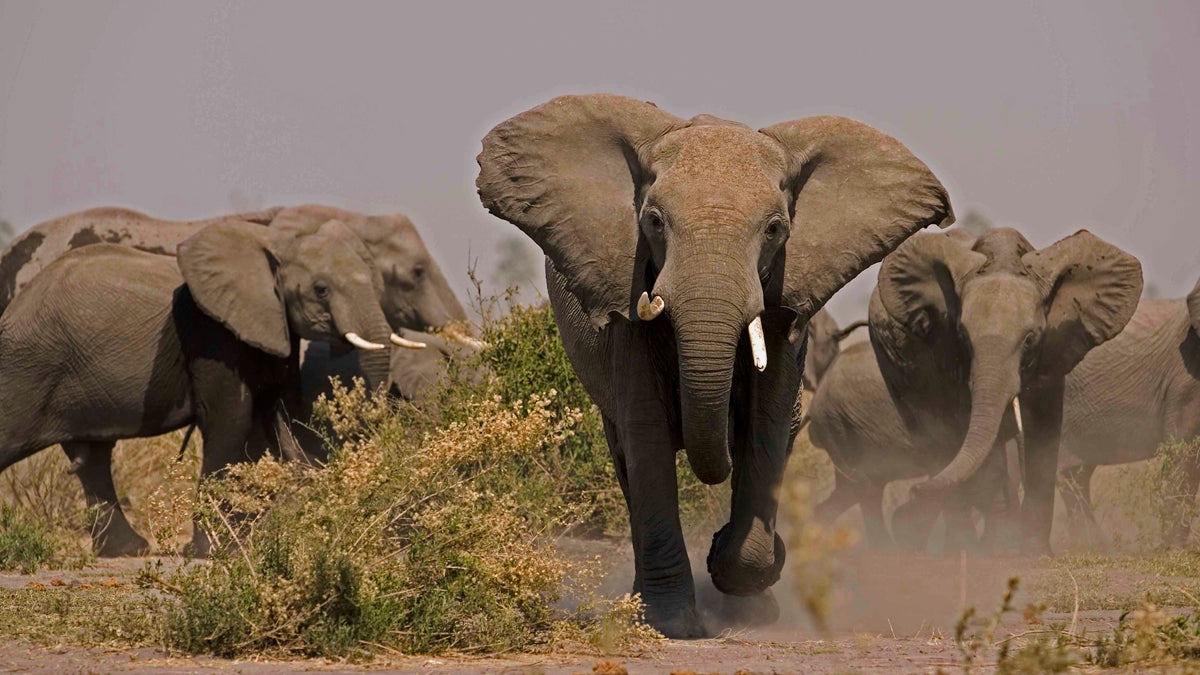The image captures a dynamic scene of wildlife, featuring a herd of elephants advancing across a savannah. Dominating the center of the photograph is a majestic gray elephant, its large ears extended wide and its tusks gleaming white. This central elephant strides directly towards the camera, its powerful legs in mid-motion, accentuating the sense of movement. Surrounding it are several other elephants, some following from the left to the right, while others appear further in the background, contributing to the depth of the scene. The ground beneath them is a mix of bare dirt and sparse, dry shrubs with green bases and yellowing tips, indicating a harsh, semi-arid environment. A noticeable cloud of dust rises from the earth, kicked up by the elephants' march, enhancing the lifelike action captured in the photo. The sky overhead is hazy and light gray, casting a subdued, almost monochromatic tone over the landscape. The overall effect is a vivid portrayal of these magnificent creatures in their natural habitat, marked by a blend of earth tones and the occasional shimmer of green foliage.